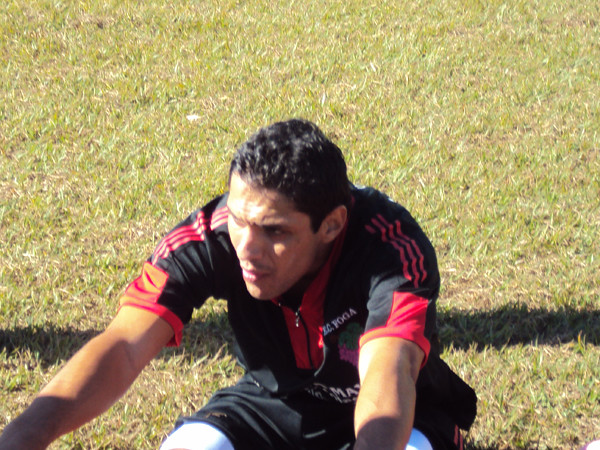In this image, we see a man who appears to be a soccer player, dressed in an athletic uniform. He is sitting on the grass and performing leg stretches, extending his legs straight out in front of him while reaching forward with his arms as if touching his toes. His attire includes a black shirt with a zipper and red accents, featuring three red stripes running down each shoulder and a red square on the sleeves near the shoulders. He also wears black shorts and white knee or shin guards. The man, who has short brown hair, is glancing off to his right. The scene is brightly lit by the sun, casting a strong light and creating distinct shadows on the grass around him, including a prominent horizontal shadow behind him. The photograph captures him mid-stretch during what seems to be a warm-up session for an outdoor sport, likely soccer.